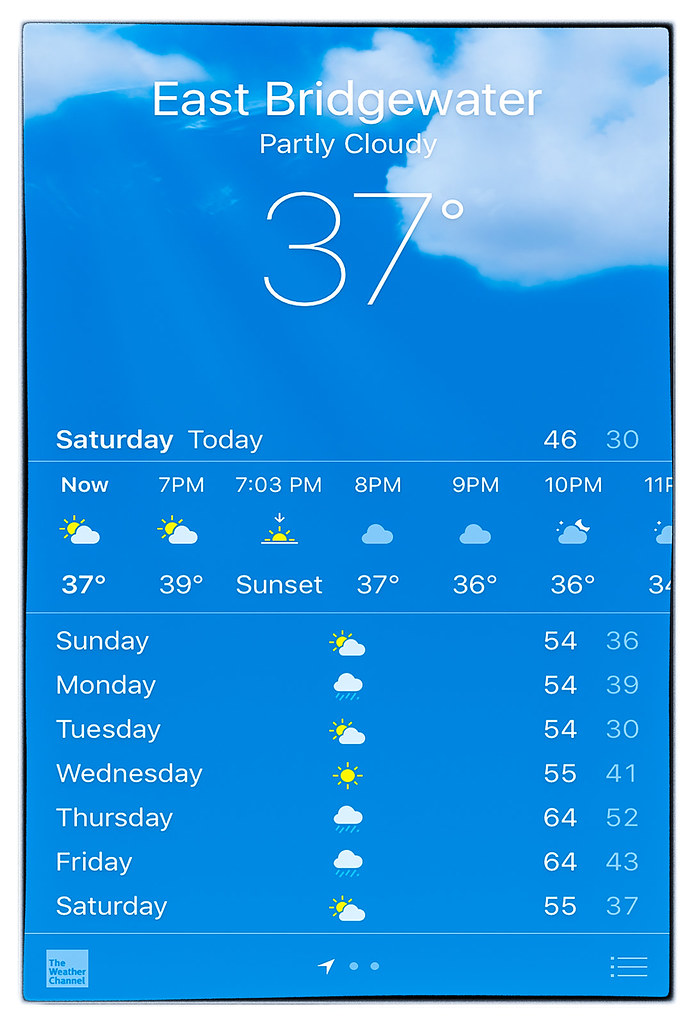This detailed caption describes a mobile screenshot from a weather app, focusing on its appearance and functionality:

---

The mobile screenshot displays a weather app interface. The background at the top of the page is a blue sky with scattered white clouds, setting a serene tone. Prominently featured at the top is the location "East Bridgewater," accompanied by a weather description "Partly Cloudy" and a current temperature of 37 degrees Fahrenheit.

Directly below this, a section outlines the hourly forecast for the current day, which is Saturday. The app provides a scrolling timeline that begins with "now," followed by specific times such as 7 p.m. (including the sunset time), 8 p.m., 9 p.m., 10 p.m., and so on. Each time slot is paired with an anticipated temperature reading.

Further down, there is a seven-day forecast presented in columns. Each column represents a day of the week from Sunday to Saturday, indicated by their respective abbreviations. Rows within these columns include weather icons that visually depict conditions like partly cloudy, cloudy with rain, or sunny, alongside the high and low temperatures forecasted for each specific day.

This well-organized app allows users to quickly grasp both the current weather situation and the upcoming week's forecast through its clear and efficient layout.